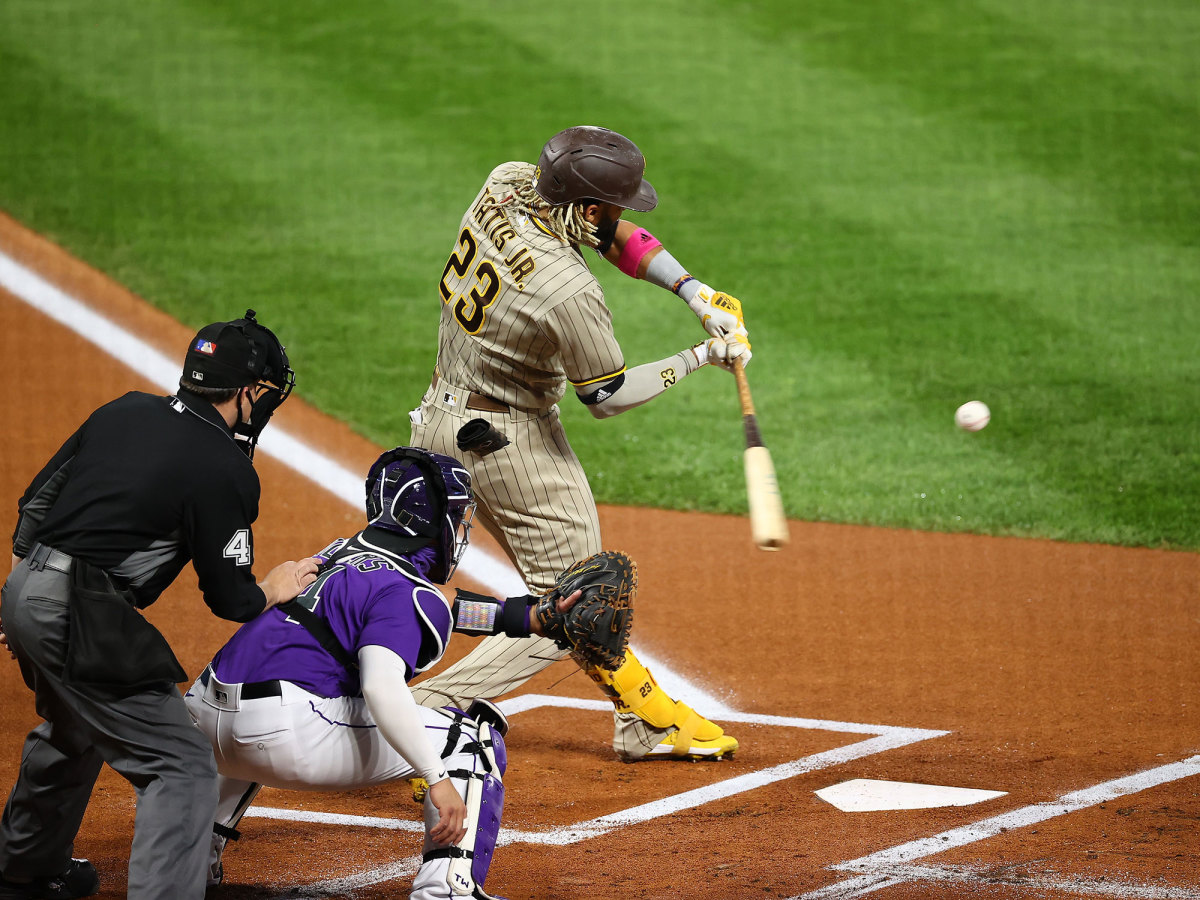In this live-action photograph of a baseball game, the intense moment captured is of a batter in mid-swing at a baseball just over home plate. The batter, adorned in a distinctive white and brown striped uniform with yellow and black letters, is wearing a black helmet from which strands of hair emerge at the back. His cleats are bright yellow, adding a splash of color to his outfit. The bat he's wielding is white, transitioning to black towards the handle, with a brown base. 

Positioned behind him are the umpire in a black outfit, marked with a number 4 on his right arm, and the catcher, clad in a blue jersey and a catcher's mask, with his left arm extended, ready to catch the pitch. Though the bat and baseball are slightly blurred due to the motion, their positions are distinct, emphasizing the fast-paced action of the moment. The well-maintained field with its green grass, perfectly lined batter's boxes, and home plate provide a picturesque backdrop for this intense play. The zoomed-in focus on the players accentuates the high energy and anticipation of this critical game moment.